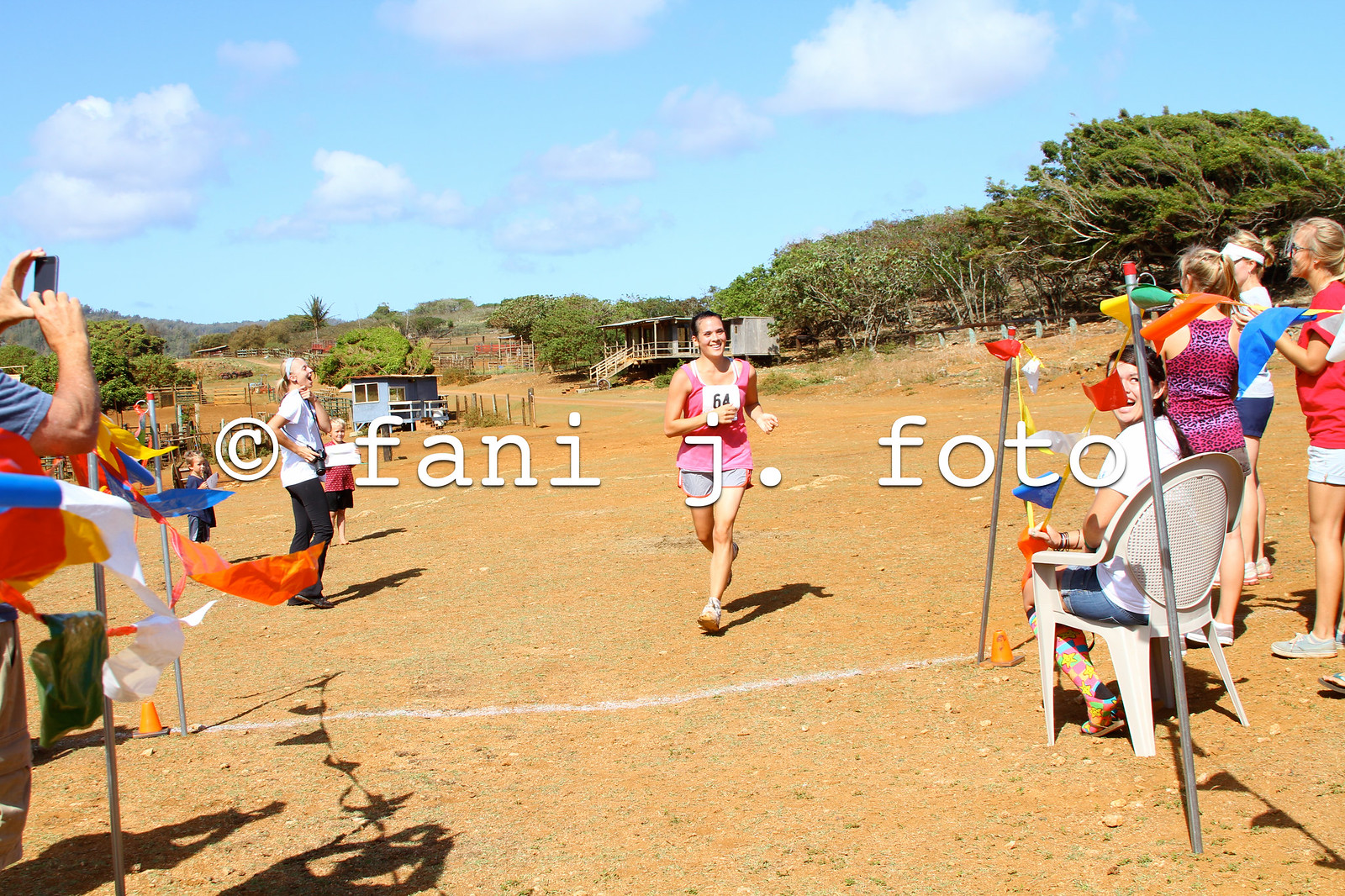In this captivating photograph, a joyful female runner clad in a bright pink tank top and gray shorts with red borders, marked with the race number 64 on a white placard, is seen sprinting towards the finish line. She is sporting white sneakers and has her dark hair tied back as she beams at the small crowd eagerly assembled at both sides of the finish line. The finish line itself is demarcated with a white chalk line flanked by metal poles adorned with colorful flags and tassels. The path is lined with dirt and small rocks, creating a rugged terrain typical of a subtropical or sub-arid landscape. Behind the cheering onlookers, who are snapping photos and clapping, an array of small, rustic houses built on stilts and scattered scrub-like trees extends into the background under a bright blue sky dotted with fluffy white clouds. A visible watermark in large white letters reading "FANI J.FOTO" signifies the photograph’s copyright.